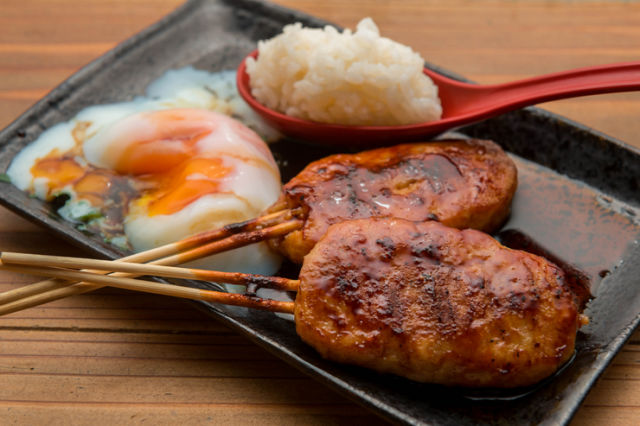In this photograph, we see a neatly arranged meal presented on a black, rectangular tray positioned diagonally on a dark, wooden table that almost resembles bamboo. The dominant feature is a red, deep serving spoon filled with a dome of white rice, centrally placed towards the top. On the bottom right of the tray, there are skewers with rounded patties of meat, possibly pork, beef, or chicken, featuring evident grill marks and a reddish-brown hue from a barbecue sauce. To the left, there's a split over-easy egg with the yolk intact but slightly exposed, giving a visual hint of its runny interior. The entire setup creates an appealing, detailed presentation on the tray.